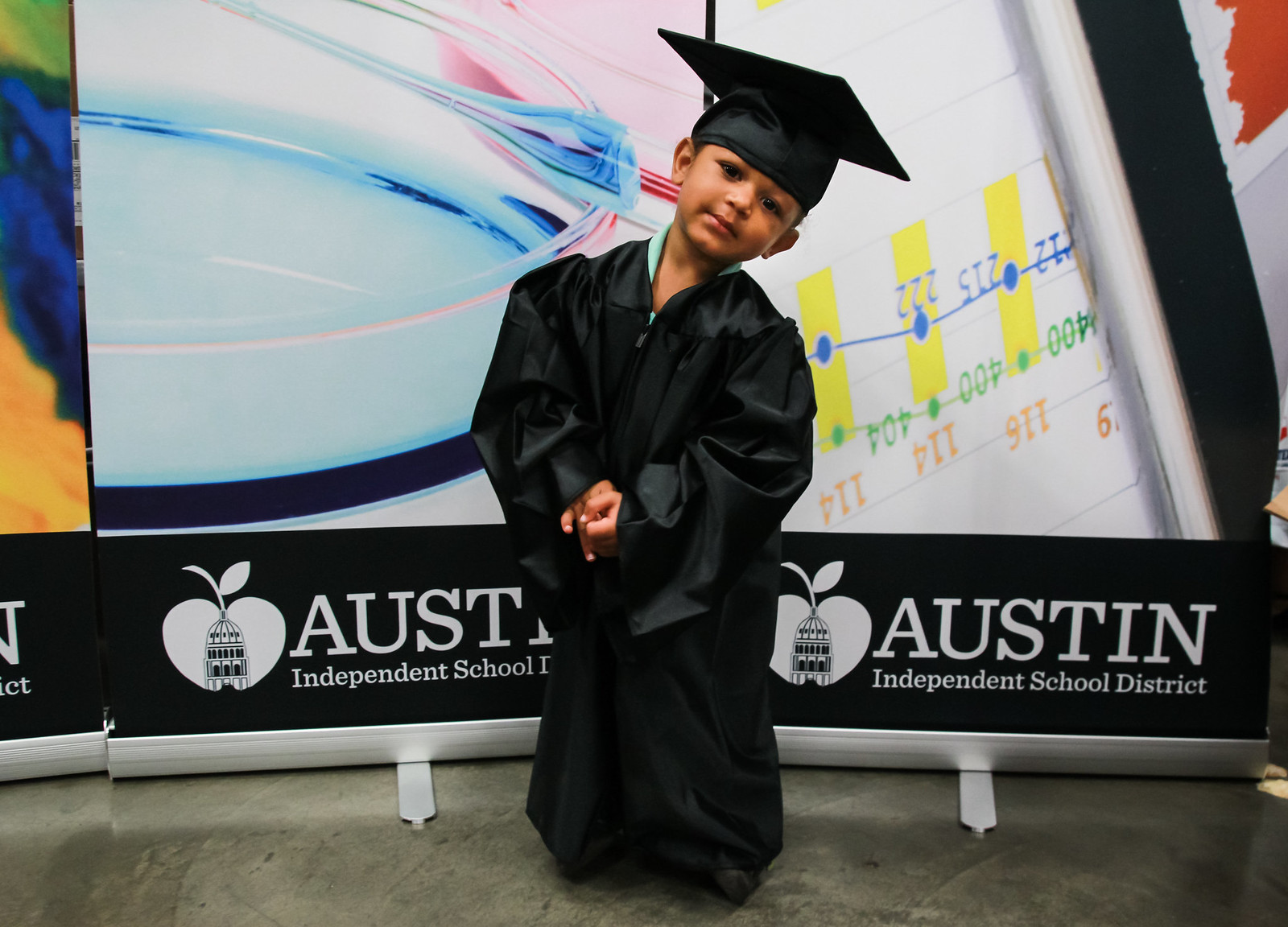In the photograph, a young boy, around four to six years old, is the central figure, standing and wearing a light green shirt partially covered by a silky black graduation gown and matching cap. His head is tilted slightly to the left, and he gazes at the camera with a slight smile. In the backdrop, a banner prominently displays "Austin Independent School District" in white letters against a black background. Adjacent to the text is a white apple icon superimposed on a dome-topped building, resembling the Capitol. The surroundings include an array of colorful elements: a dominant swirly blue-and-white design, a large purple-blue section, yellow splotches below it, and an intricate mix of numbers such as "400" oriented upside-down along a green line. A vertical black bar runs along the top right to the bottom right. The floor in the image has a gray tone, and additional background details include what appears to be lab equipment and bar chart features. An orange splotch is visible in the upper right corner, adding a touch of vibrancy to the scene. There are no other people in the photograph, and the overall color scheme consists primarily of black, white, blue, and red.